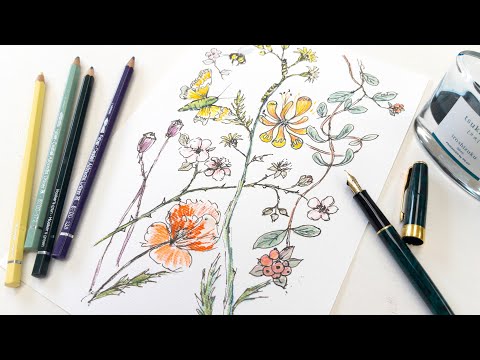The image depicts a flat lay photograph of an artist's work table. Central to the image is a white sheet of paper, slightly tilted to the right, showcasing a detailed colored pencil drawing of various flowers and butterflies. The drawing includes vibrant florals such as an orange iris-like flower with a green stem in the lower-left corner, pink rosebuds, white five-petaled flowers, and small red and orange blossoms. A bright yellow butterfly with green body rests prominently on the left side of the central yellow flower.

Adjacent to the drawing are art supplies laid out on the desk. To the left of the paper, four colored pencils are neatly aligned horizontally in the shades of yellow, green, black, and blue. On the right side, a sophisticated green fountain pen with gold accents is placed at a 45-degree angle, its black lacquer cap with a gold band beside it. Additionally, there is a clear glass ink bottle whose label is not fully legible, suggesting it might be in a foreign language. An unknown silver object is also slightly visible in the upper right area of the photograph.